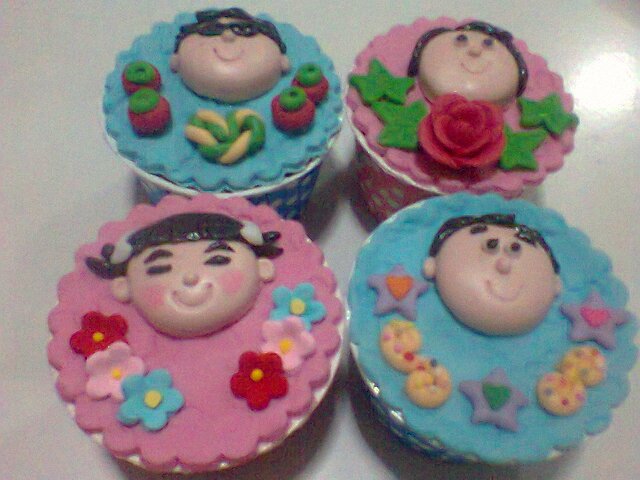The photograph features four intricately decorated party favors or handmade gifts, resembling cupcakes or small containers, each made with a high level of detail. These favors are arranged in a pattern with teal blue and pink alternating colors—top left is teal, top right is pink, bottom left is pink, and bottom right is teal. The containers, which are about the size of muffin cups, are topped with scalloped-edge felt lids adorned with multi-colored, finely detailed felt cutouts and stitching. Each lid features a child’s face, made to look like either a doll or cartoon character.

There are two boys and two girls represented. The boy in the top left has black hair and is wearing black glasses. The girl in the top right has short brown hair without additional adornments. The girl in the bottom left has rosy cheeks, eyebrows, and barrettes in her hair. The boy in the bottom right has short brown hair without glasses. All the faces have black hair and are decorated to resemble Hispanic children. The detailed embellishments on the lids include flowers, leaves, stars, and intricate swirls, mimicking frosting decorations. The decorations and the festive color choices of aqua and pink make these favors both colorful and visually appealing, highlighting fine craftsmanship and a playful, child-friendly theme.